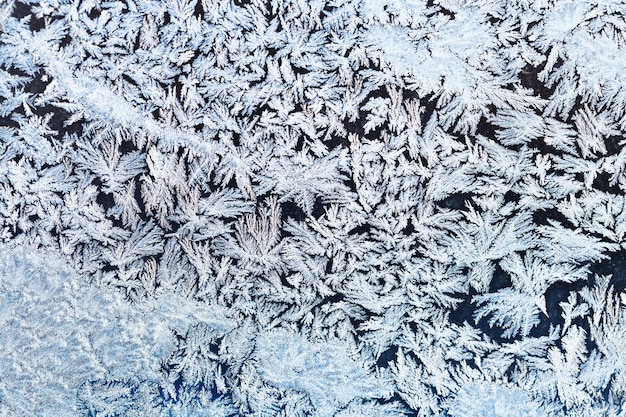The image, likely a close-up photograph taken under a microscope, depicts an intricate and delicate scene of ice crystals that closely resemble fern leaves or snowflakes. The background is predominantly black, adding a stark contrast to the predominantly white frost patterns. Towards the bottom left and right corners, there is a subtle blue tint, enhancing the visual depth of the scene. The ice crystals fan out in intricate, feather-like patterns, showcasing a variety of unique shapes and structures. These crystalline patterns are densely packed in some areas, particularly towards the edges and corners, giving the impression of a frosted glass surface viewed on a typical winter's day. The textures are multifaceted, ranging from solid icicle blues to softer whites, creating a harmonious blend that fills the entire frame. The overall appearance is both delicate and complex, evoking a sense of frozen beauty akin to a natural, frosted landscape painted on glass.